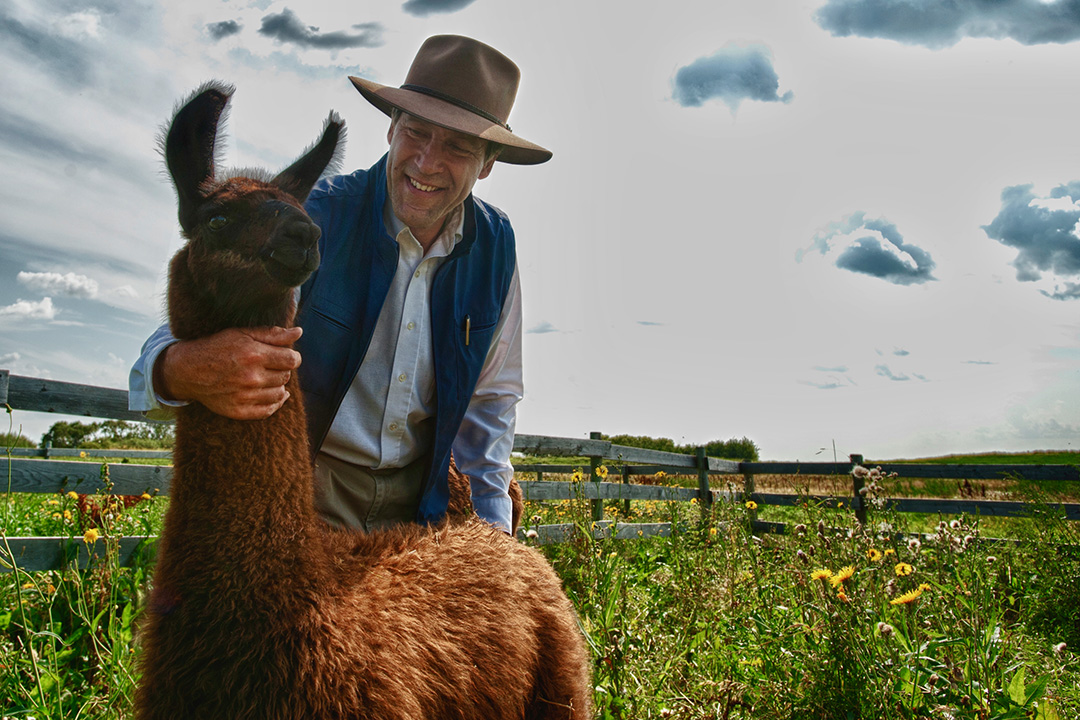In this professionally taken photo, a serene meadow, possibly farmland, stretches into the background with a light gray wooden fence enclosing the scene. The meadow brims with vibrant plants and vegetation, showcasing yellows, whites, and a touch of red flowers among the tall weeds. Central to the image is a joyous man in his fifties, dressed in a wide-brimmed brown hat, a buttoned-down white shirt, a blue vest with a pin in the pocket, and khaki pants. He is affectionately hugging a dark brown, furry alpaca with a long neck and prominent ears. The man is smiling warmly, looking adoringly at the alpaca as he tenderly pets it. Above, the sky is a bluish-gray, filled with dark clouds that hint at imminent rain, though sunlight still peeks through, illuminating the tranquil bond between the farmer and the alpaca.